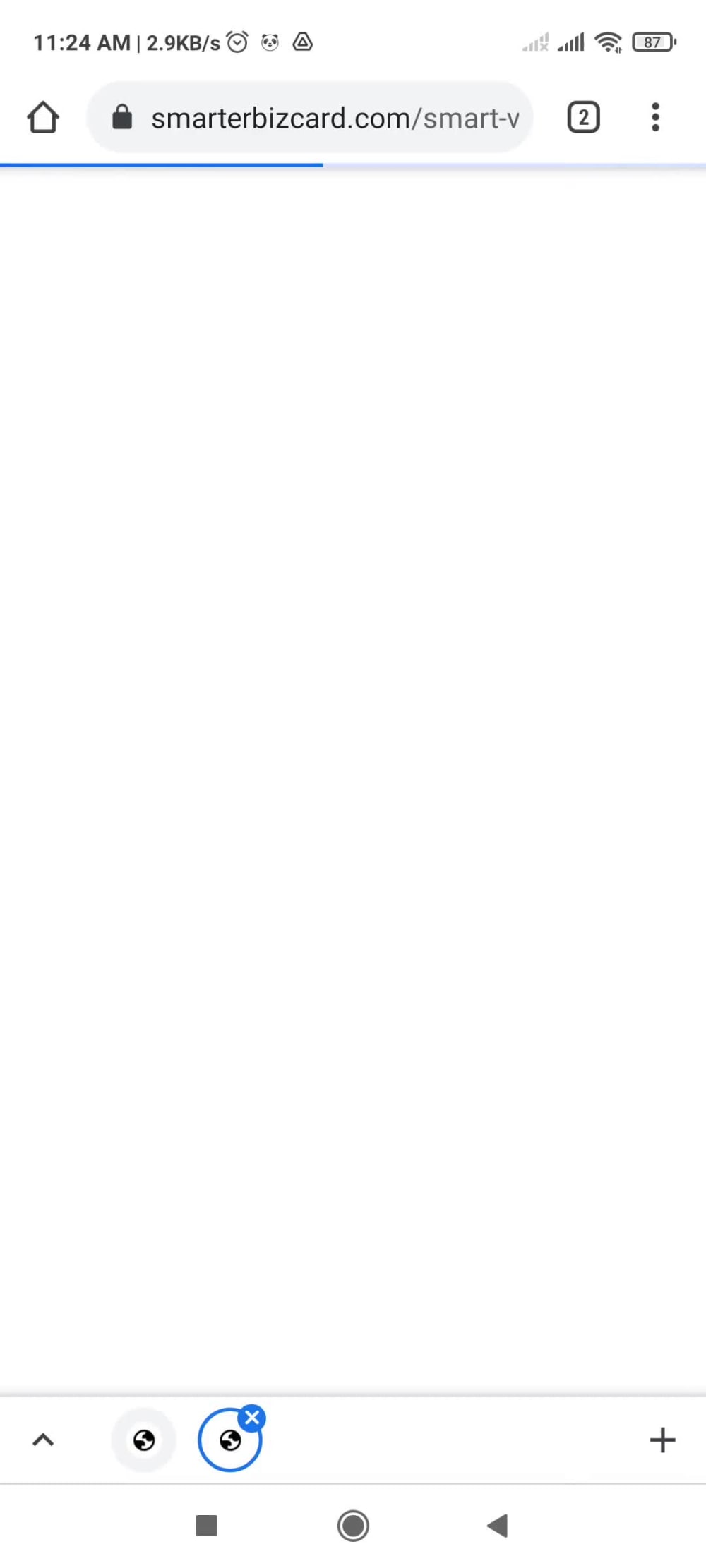A detailed screenshot of a mobile device taken at 11:24 a.m. The screen displays full carrier signal strength, a fully connected Wi-Fi signal, and a battery life at 87%. Various status icons are visible, including an alarm clock, a panda, and a data rate of 2.9 kB/s. The device shows a home icon with a white background and black outline.

The browser is open to a secure website, smarterbizcard.com, indicated by the locked web address icon. There are two open tabs, denoted by the "2" next to the tabs icon, and a vertical ellipsis (three-dots) for more options. A blue progress bar runs across the top of the page. 

The bottom of the screen features a white, empty app space with several icons: an up arrow, a globe, a secondary globe enclosed in a blue circle with an "X" on it, and a plus sign to the far right. Additionally, play control icons are visible at the bottom, including stop, record, and rewind buttons.